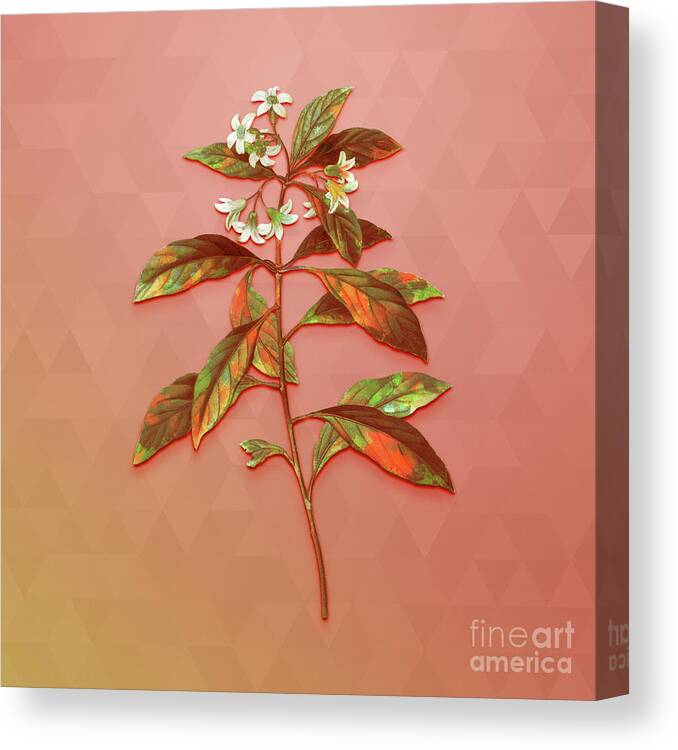In this detailed photo, a slender plant branch is set against a peach-colored, geometrically patterned background with small triangles. The central stem, which is thin and upright, features alternating leaves in shades of green, orange, brown, and some yellowing. Notably, the leftmost bottom leaf appears to be partially eaten. At the top of the stem, approximately ten tiny white flowers, each with a green center, are clustered on small brown stems. The image is framed in a rectangular shape, reminiscent of a picture box cover, and in the bottom right corner, it bears the text "fine art america" in lowercase white letters.